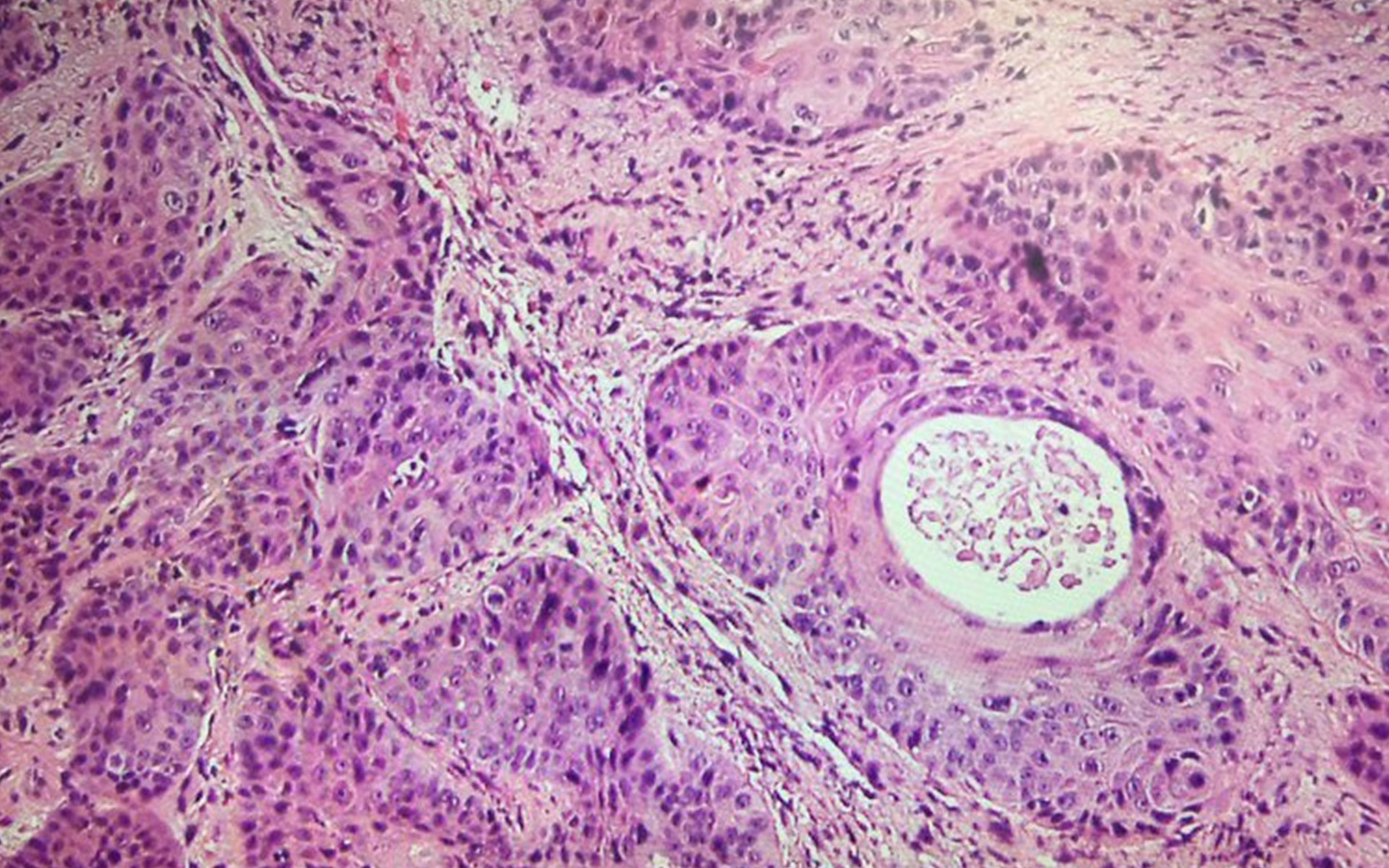This detailed close-up photograph, appearing to be a scientific slide or sample, resembles a vibrant painting with its rich palette of purples, pinks, and whites. The image, likely captured under a microscope, features an array of intricate patterns and textures that create an almost three-dimensional effect. Predominantly adorned in pale pink and accented with darker pinks, mauves, and purples, the composition is both mesmerizing and complex. On the right-hand side, a distinctive white, uneven circular feature stands out, potentially representing a cell or tumor tissue. This focal point, dotted with smaller purple circles and lines, adds to the overall perception of biological intricacy. The scene may depict muscle, blood, or organ tissue, inviting viewers to ponder the exact nature of the sample. The interplay of colors and shapes makes the photograph not only scientifically intriguing but also artistically compelling.